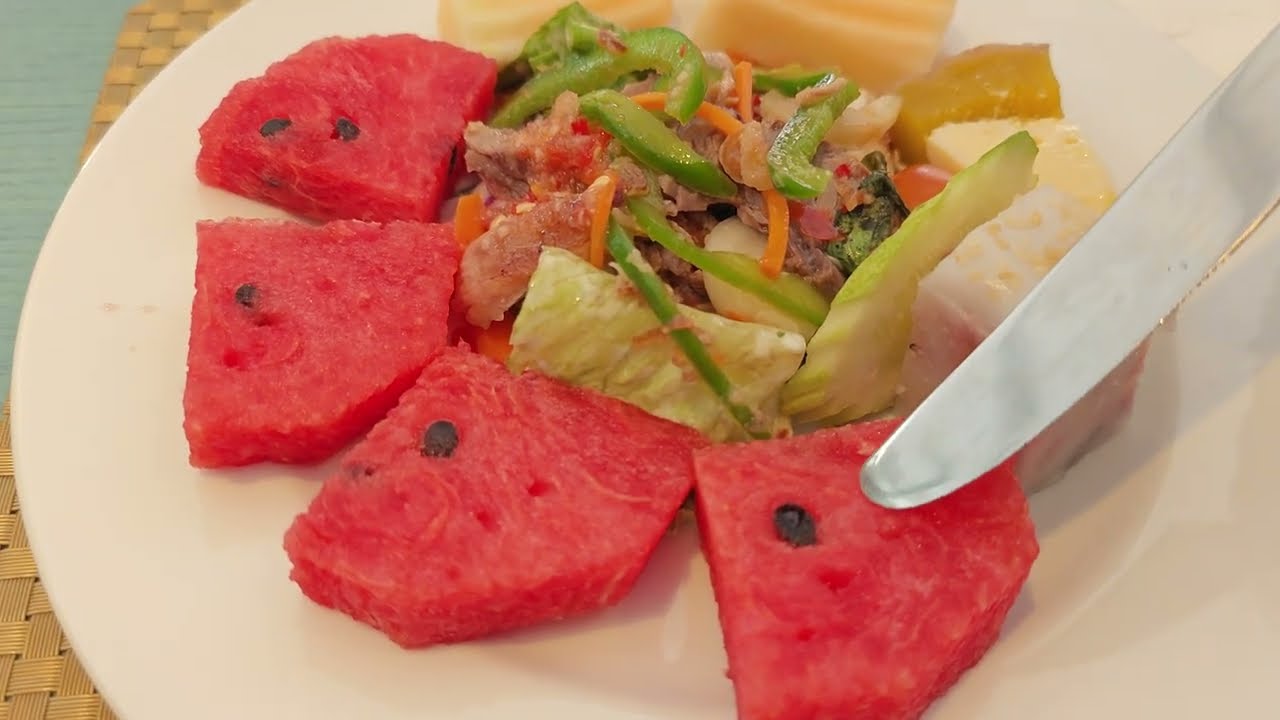The photograph captures a close-up of a white round plate placed on a brown wooden basket-weave placemat atop a green table. Surrounding the inner contents of the plate, which primarily consists of a mixed green vegetable salad, are four pentagon-shaped slices of watermelon, each edged with distinct small black seeds. The salad features a variety of elements such as celery, lettuce, green bell peppers, carrots, tofu, broccoli, and possibly even some pieces of octopus. Nestled among the watermelon slices, from 12 to about 2 o'clock, are three slices of ripe cantaloupe. A curvy silver knife extends from the upper right of the photograph, its blade touching one of the watermelon slices. The intricate details of the plate, the woven texture of the placemat, and the hint of a green floor surface contribute to the overall warm and natural ambiance of the setting.